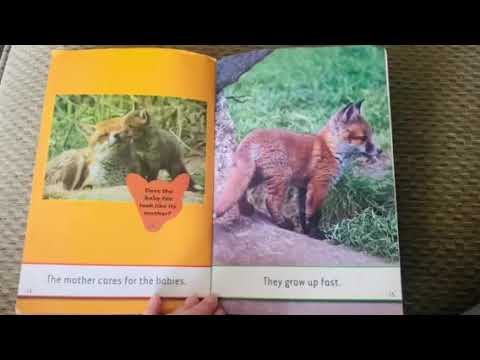The image depicts an open children's book about animals, specifically foxes, with visibly letterboxed top and bottom edges. The left page, against a yellow background, features a central photo of an adult fox nuzzling a baby fox amidst greenery, and contains an orange-colored text framing the image. At the bottom, it reads, "The mother cares for her babies." The right page showcases a solitary baby fox standing in the grass and partially on a concrete area, with the fox facing towards the right. This page has a complementing textual note at the bottom stating, "They grow up fast." Both pages are held open over a light brown fabric or couch by a visible Caucasian hand positioned at the lower center, primarily showing the tips of the fingers. The overall color palette of the scene includes yellow, green, brown, and white.